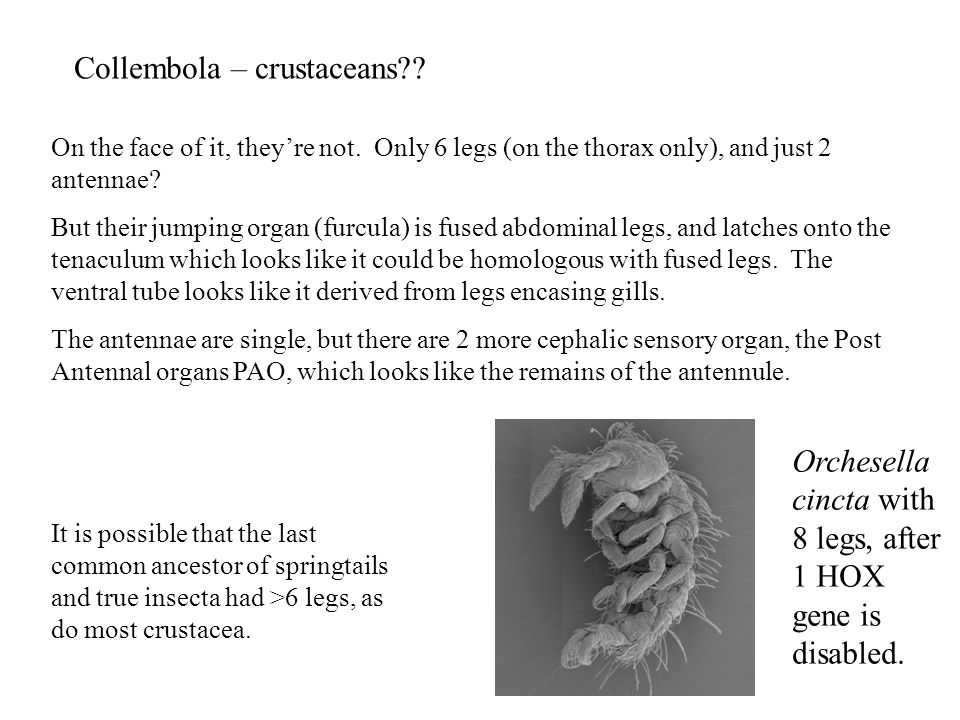The infographic presents black text on a white background, featuring dense academic content about Collembola (springtails) with a speculative connection to crustaceans. At the top, bold text reads "Collembola-Crustaceans?", hinting at the debated evolutionary link between the two groups.

Beneath the heading, the first paragraph states: "On the face of it, they're not: Only six legs on the thorax, and just two antennae?" It goes on to explain that their jumping organ, called the furcula, is actually fused abdominal legs that latch onto the tenaculum. This organ is considered homologous with fused legs. Additionally, it mentions that the ventral tube, an anatomical feature of springtails, seems derived from legs encasing gills.

The following section discusses sensory organs: "The antennae are single, but there are two more cephalic sensory organs, the post-antennal organs (PAO), which appear to be the remnants of additional antennae."

In the lower-left corner, another block of text theorizes: "It is possible that the last common ancestor of springtails and true insects had greater than six legs, similar to most crustaceans."

To the lower right, there is a black-and-white photograph of a small, multi-legged creature, likely with projections from its back. Adjacent to the image, text states: "Orchesella cincta with eight legs after one HOX gene is disabled."

This detailed infographic scrutinizes the morphological and genetic mysteries linking springtails to crustaceans, illustrated with an evocative image of these tiny creatures.